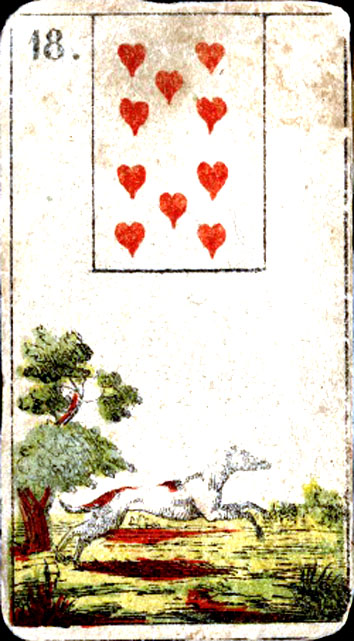This captivating image presents a detailed, vintage-style illustration with an antique charm. The artwork, characterized by its oblong shape, could either be a meticulously printed piece or a hand-drawn illustration. Notably, in the upper left corner, the number '18' is distinctly visible. Adjacent to this, there is a playing card-like image adorned with several heart symbols, though it bears no numbers.

The lower half of the image showcases a finely rendered illustration of a lean dog, reminiscent of a greyhound, depicted in shades of black and grey. The background vividly portrays a green pasture interspersed with red patches, likely representative of flowers. On the left side of the illustration, a robust tree with a reddish-brown trunk stands prominently, displaying an array of white blossoms and green leaves. These elements collectively contribute to the image’s rich, detailed aesthetic, evoking a sense of nostalgic allure.